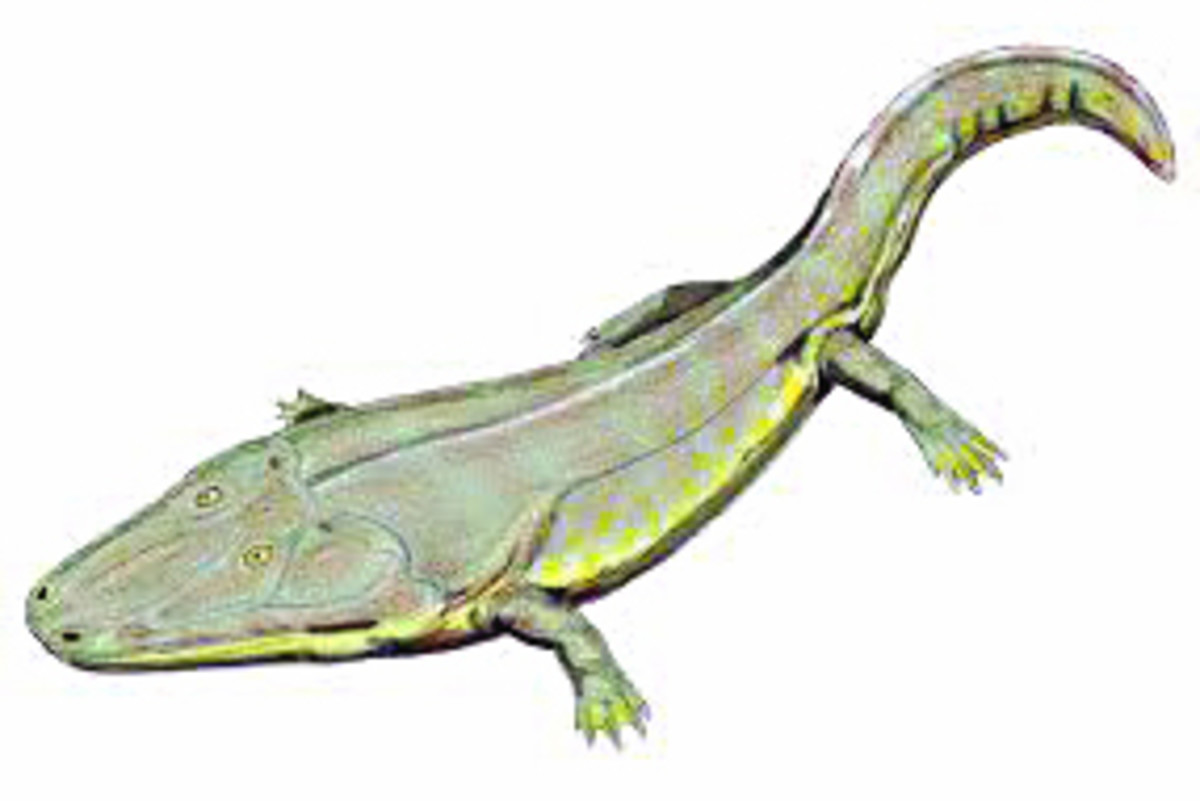This image features a hand-drawn or cartoon-style illustration of a large reptile—likely an alligator, given its rounded snout—set against a completely plain white background. The central and sole subject in the image is this alligator, distinct with its greenish skin on the top and a yellowish-green tint on its belly. The coloration is nuanced with various shades, including muted greens and whites flecked with fluorescent yellow on the belly and the webbing between its clawed feet. The alligator is oriented facing the left side of the image, with its tail slightly curved and its left arm and leg fully visible while the right limbs are partially hidden by its body. The eyes are yellow, perched on top of its head, with noticeable nostrils at the base of its snout. The overall style looks like hand-drawn artwork, possibly a digital painting, showcasing fine details like the alligator's claws, eyes, and textures on the skin.